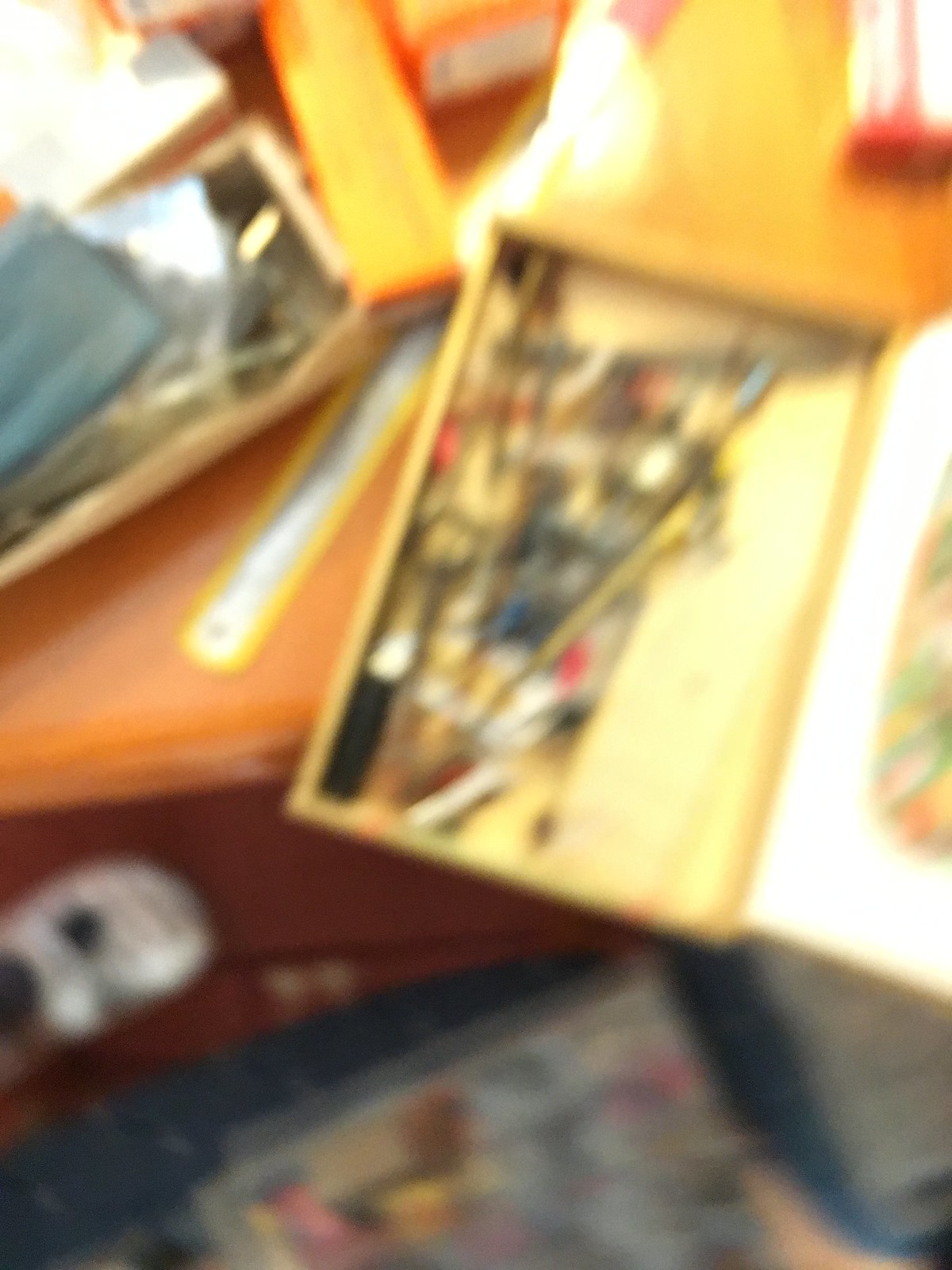The photograph is extremely blurry and out of focus, making it difficult to discern specific details clearly. At the center of the image, there appears to be a yellow box or perhaps a yellow toolbox with a hinged lid, resembling a cigar box, sitting on a wooden table or desk. The inside of the box seems to contain various small items like pins, screws, trinkets, or tools such as paintbrushes or doorknobs. Surrounding the main box, there are other open-top containers filled with what looks like tools or similar items. Near the bottom left of the image, there is a shape that resembles a person's foot with two sandal straps. On the floor, there's something that looks like a magazine featuring pink, yellow, and light blue colors. Additionally, a desk lamp appears to be illuminating the scene. The background includes vague impressions of concrete or gray surfaces and possibly some envelopes lying on the desk. The floor beneath the desk/workstation looks wooden and cluttered with various objects.